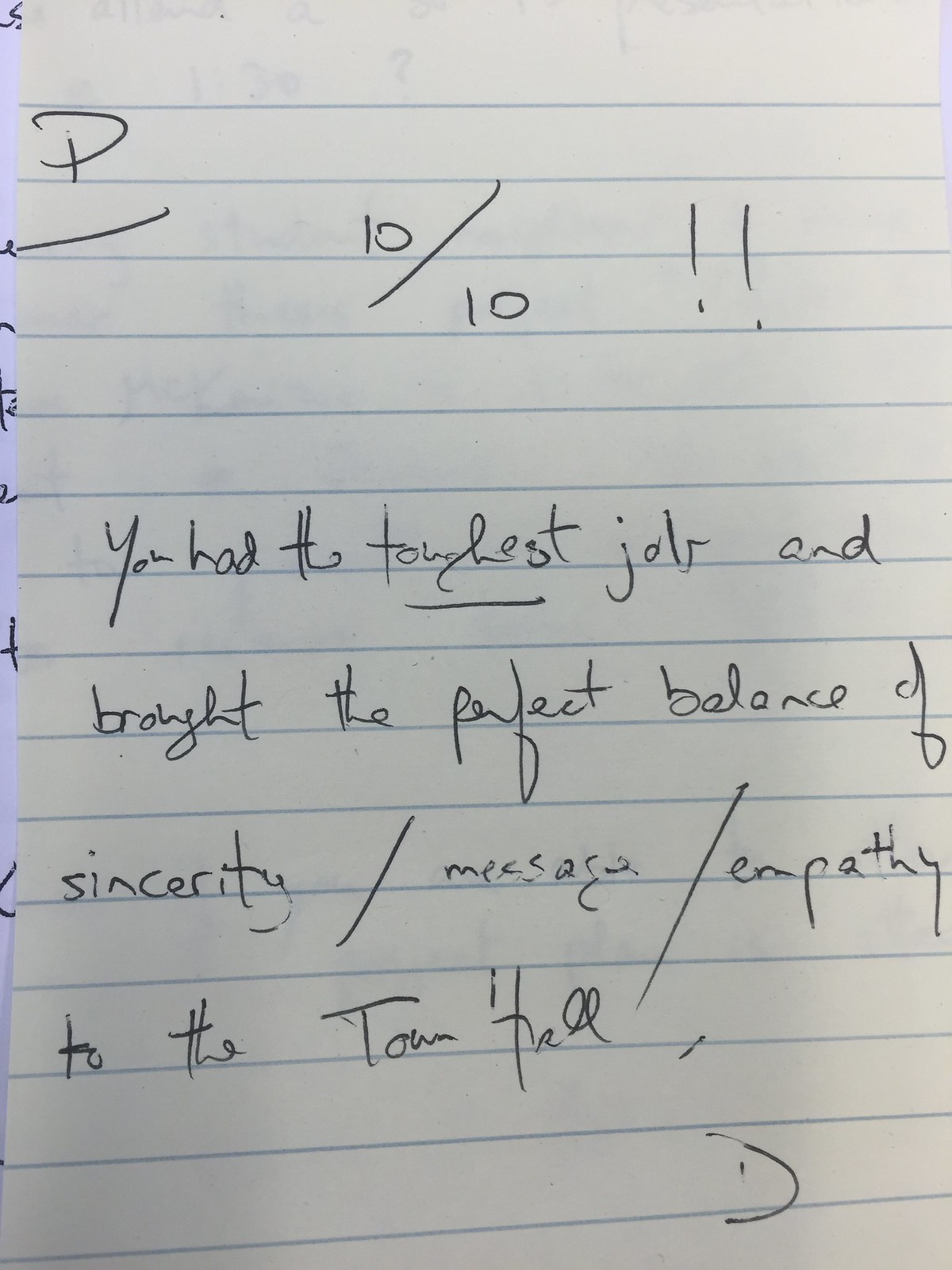This appears to be an image of a graded handwritten note on wide-ruled notebook paper with light blue lines. The paper is written in black ink and features a variety of annotations. In the upper left corner, there is an underlined letter "P." At the top center of the page, "10/10!!" is prominently written, indicating a perfect score. Below this score, there is a handwritten comment: "You had the toughest job and brought the perfect balance of sincerity/message/empathy to the town hall." Despite the somewhat sloppy handwriting, the message is clear. In addition, the letter "D" is signed at the bottom right corner of the page, suggesting it might be from the evaluator or grader. Overall, this image showcases a well-graded assignment, likely praising the student's excellent performance and effort.